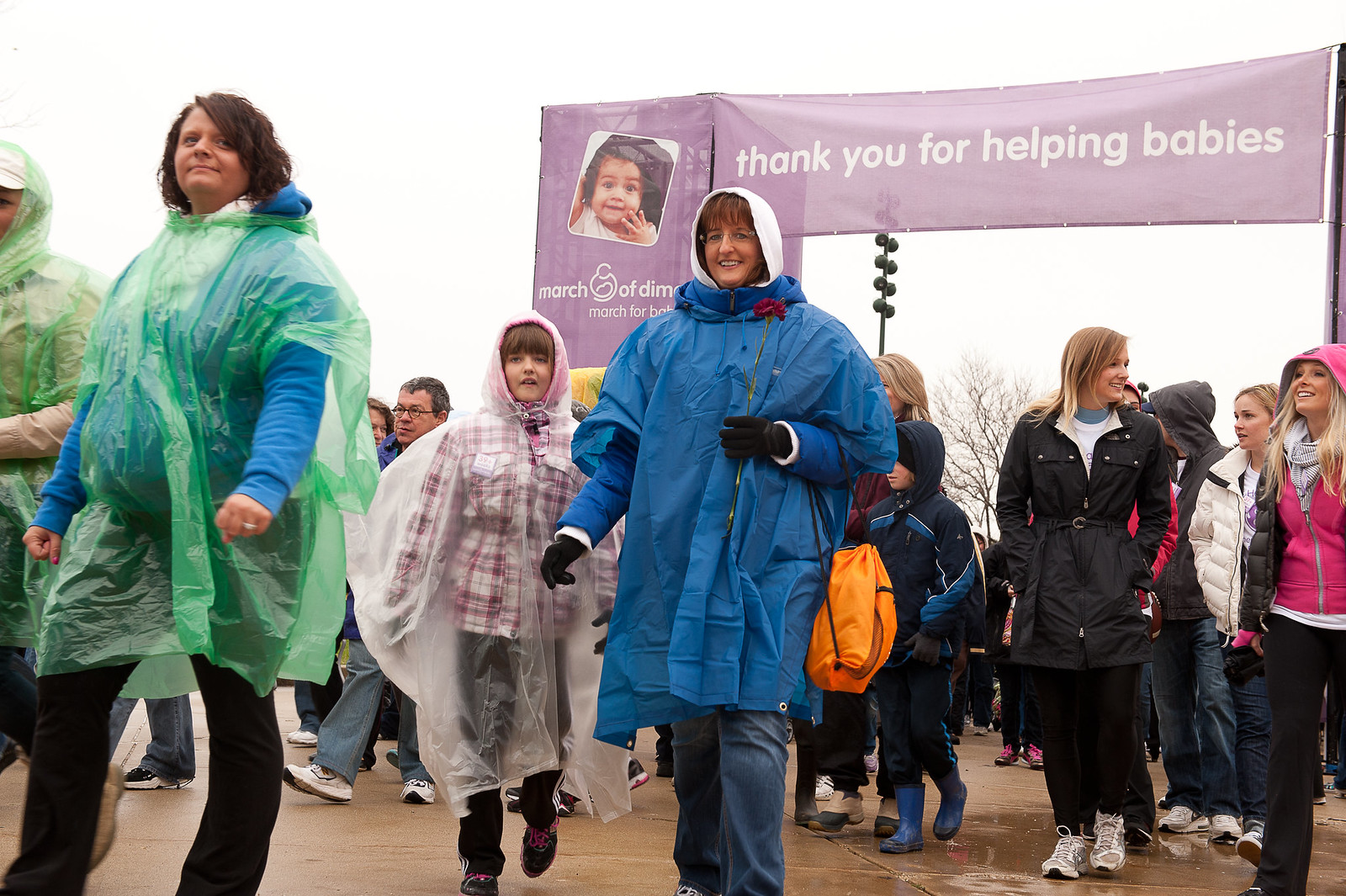The image depicts an outdoor charity walk in support of the March of Dimes. Prominently featured is a large purple banner with white text reading, "March of Dimes. Thank you for helping babies," accompanied by a small photo of a baby on the left side. The scene, which shows a drizzly, overcast day, reveals wet pavement and participants donned in various rain gear. Most of the walkers are women, with a few men scattered among the group. In the foreground, a woman clad in a large blue raincoat with a hood and an orange bag on her arm stands out. Beside her, a little girl wearing a plaid shirt underneath a clear poncho is visible. Another woman, wearing a green poncho, walks in front of them. A man in gray pants, white tennis shoes, and glasses is also part of the group. The atmosphere is determined and supportive, with many participants dressed in colorful raincoats, ensuring they stay dry during the charitable march.